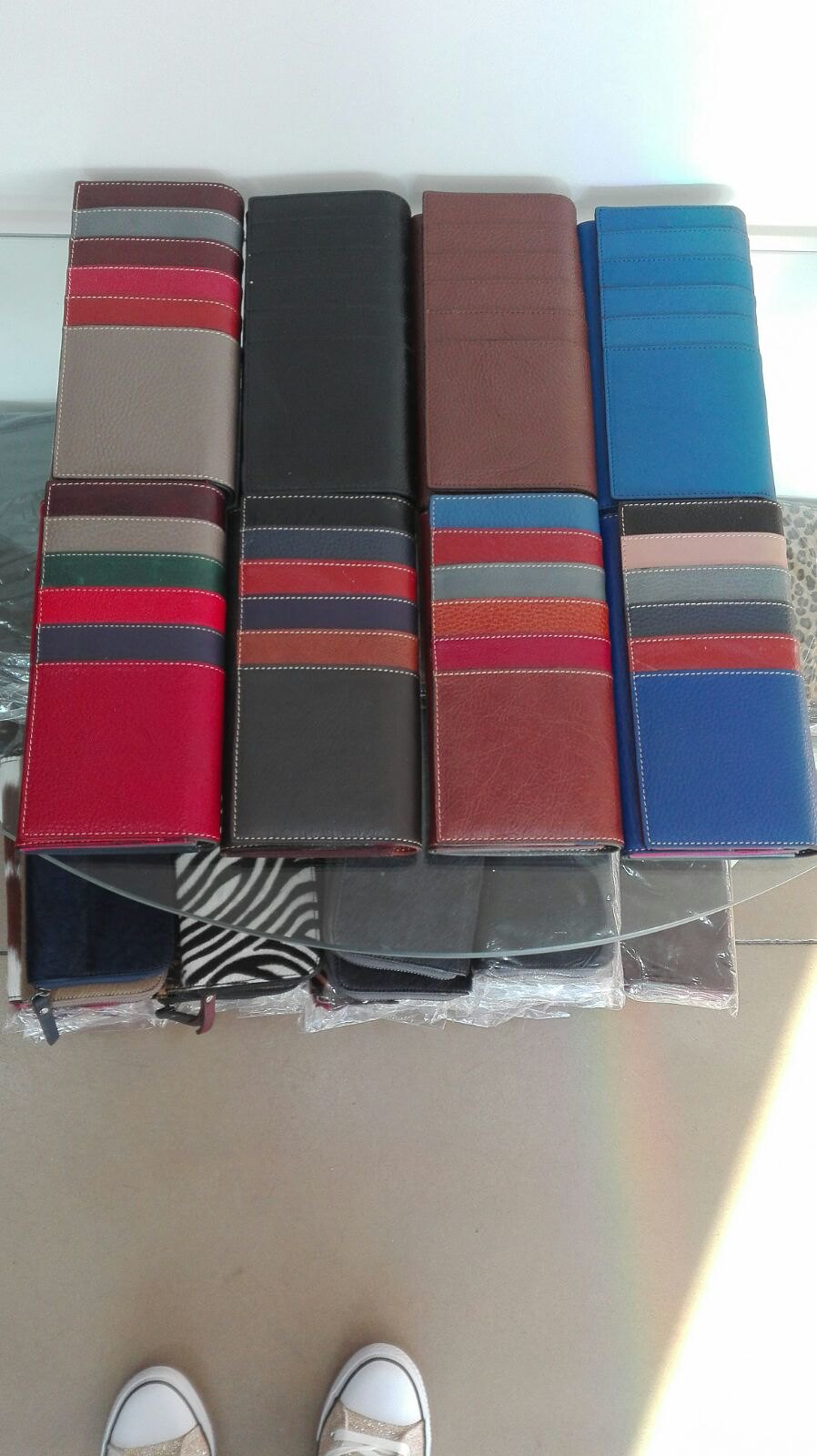The photograph features a display of various wallets on a semi-circular, glass table that is suspended off a wall. The image, captured from above, includes the photographer’s white Vans visible at the bottom left of the frame against a light brown floor. The translucent glass table holds eight wallets, prominently showcasing their unique designs; each wallet is divided into two distinct sections – half solid color and the other half adorned with multicolored stripes, suggesting compartments for individual cards.

The wallets on the table cover a range of colors, including solid black, brown, and a bluish hue. The clarity of the glass allows a view of more wallets beneath the table, which are still in their cellophane wrapping, indicating they haven't been used or opened yet. These wallets display an array of colors and patterns, such as zebra print, blue, gray, and brown.

The setting appears well-lit, possibly outdoors due to the strong sunlight reflected on the glass, which casts pronounced shadows and brightens the corners of the image. The overall background features a stark white tone contrasted by darker shadows. The image not only captures the variety of the wallets but also emphasizes the industrial-chic aesthetic of the glass table and the play of light in the scene, making it a compelling representation likely intended for product promotion.